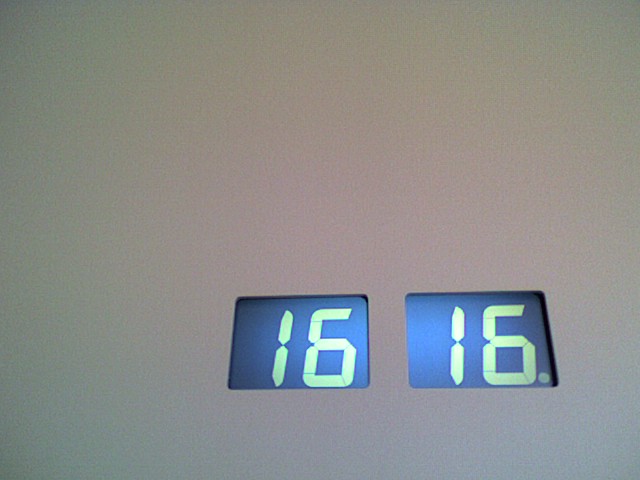A bright, white background underscores the sleek, modern aesthetic of this photograph, which features a digital display prominently situated at its center. The display, either an LED or LCD screen, showcases precise, green-tinted digital numbers that likely represent time or scoring metrics. Adding to the futuristic allure, the lower right corner of the screen is adorned with two illuminated blue squares. Each square contains a digital readout from 1 to 6, rendered in the same green digital style, further emphasizing the high-tech, streamlined design of this timekeeping or scoring device. The surrounding surface, either white or silver, contrasts sharply with the illuminated elements, making the digital numbers stand out with striking clarity.